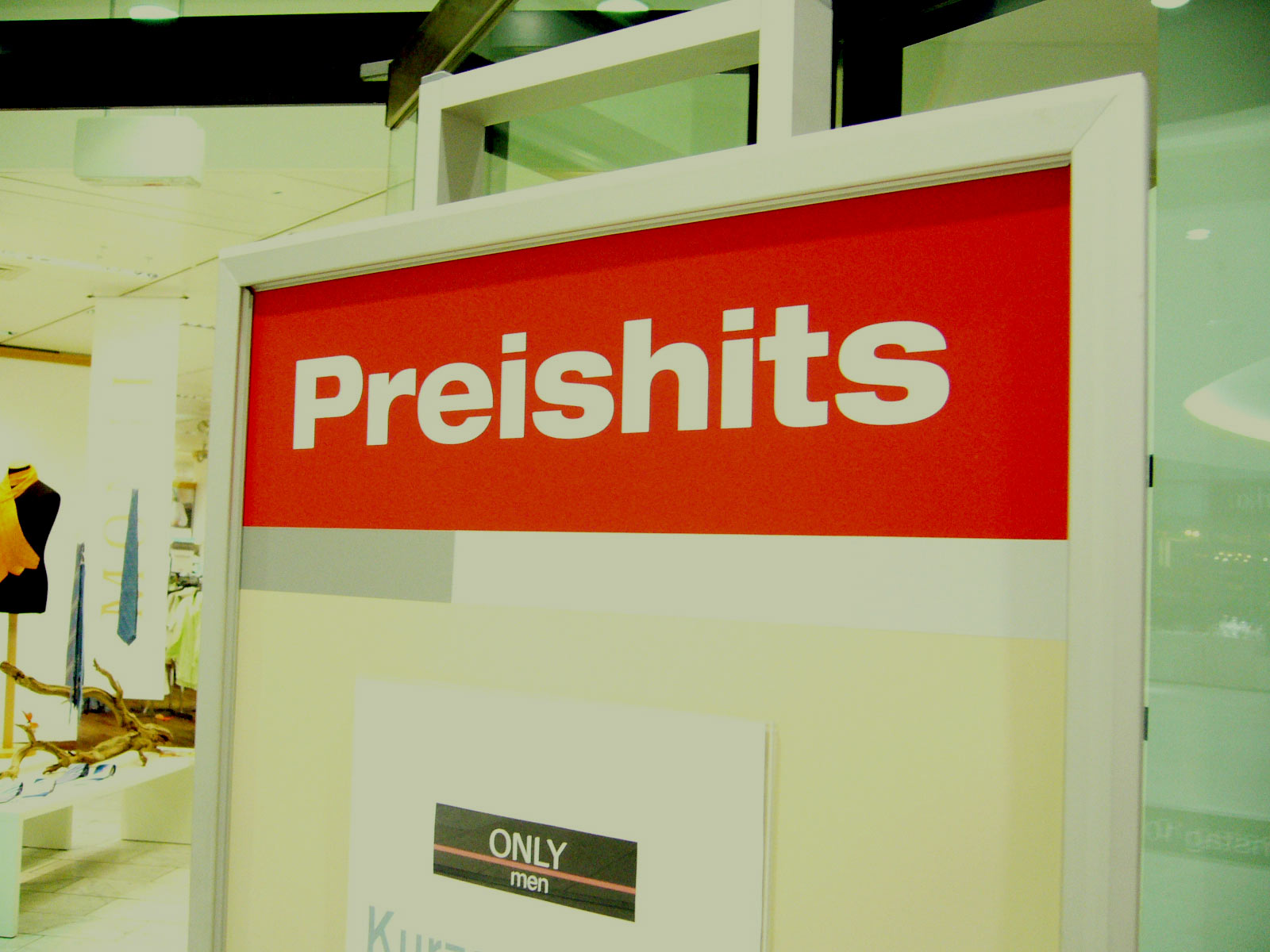This image appears to be an artist's rendering, expertly executed to mimic a realistic scene. The focal point is a close-up of a sign with bold red background and large white block letters spelling "PREISHITS," suggestively a foreign term. Below this, within a white rectangle, a black sub-heading reads "only" followed by a line, and beneath that, it states "men." This indicates the sign's specific reference to men.

In the background, the glass façade of a storefront is visible, hinting at a retail environment. To the left, a half-mannequin adorned with a scarf around its neck is positioned, with various men's ties displayed nearby, adding context to the men's fashion theme. The meticulous detailing, from the textures to the precise lettering, all suggests that this image is a painterly representation or a digital graphic rendering rather than a photograph.